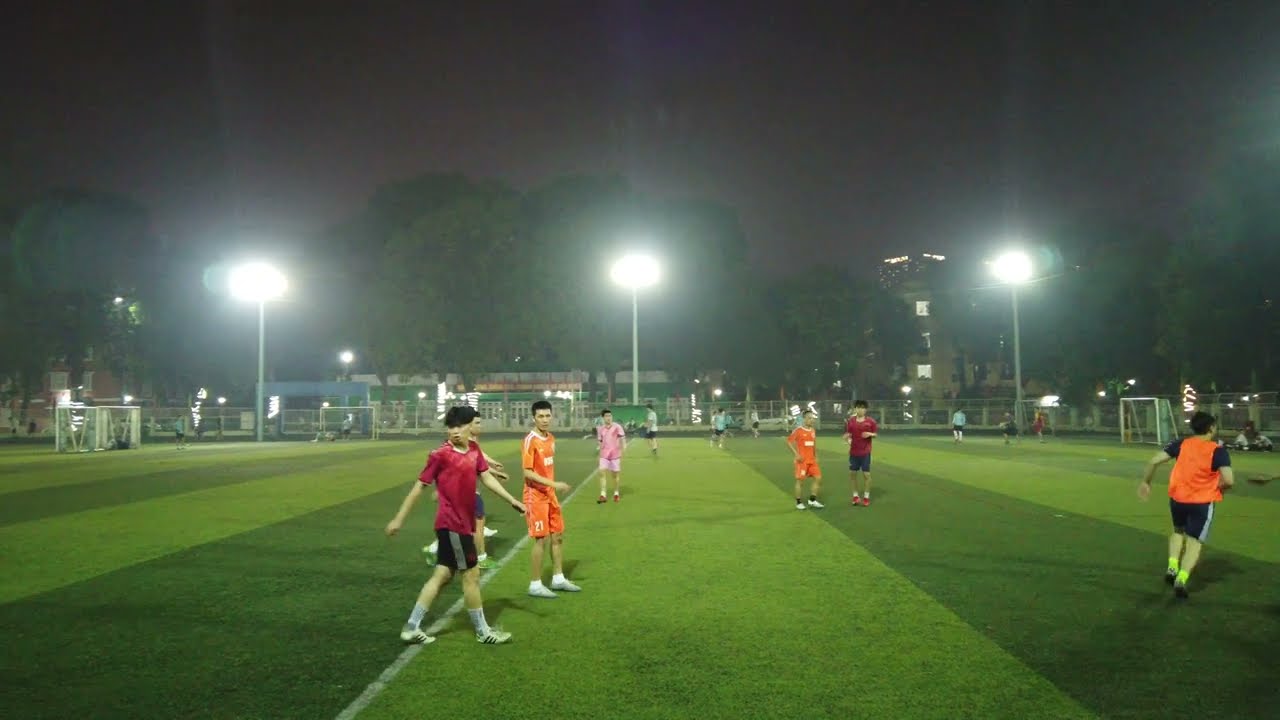This nighttime photograph captures a youth soccer game featuring teenage boys, likely around 14 years old, playing on an outdoor field. The lush green grass of the field is patterned with alternating lighter and darker lines, creating a striking visual effect. Three large stadium lights spaced evenly across the far end of the field illuminate the scene. On the right side, a white soccer net can be seen, while various players in orange, red, blue, and even one in a pink jersey, are scattered around the center of the image. Although the players appear to be standing or walking casually, the colors of their uniforms and the presence of the goalposts suggest an ongoing game. In the background, tall, leafy green trees tower over green and brown buildings, their details somewhat obscured by the resolution and the bright lights. The sky is black, confirming the nighttime setting.